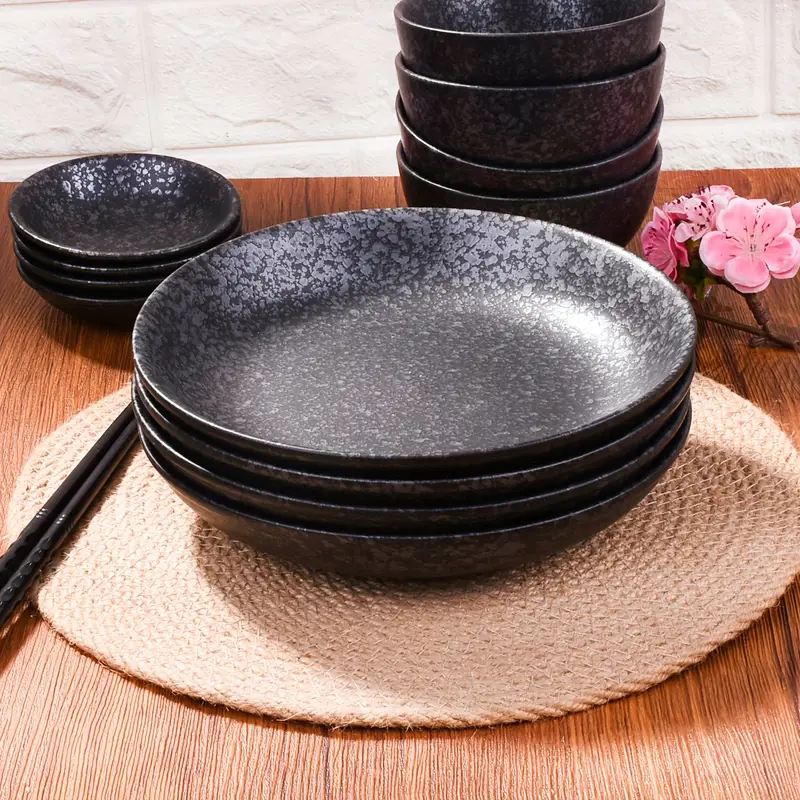In this image, set against a dark backdrop, a beautifully arranged table showcases an elegant dining set. A brown wooden table serves as the base for a round wicker placemat at the center, displaying four shallow, black marble-textured bowls stacked neatly. To the back left, a set of four smaller black saucers, also with a marble-like finish, are arranged. Directly behind the centerpiece are four deeper black bowls stacked on top of each other. Complementing the setting, a pair of black chopsticks with silver rings rest to the left side of the central bowls. Adding a touch of natural beauty, a branch with delicate pink flowers graces the right side of the table, enhancing the overall display with a soft floral accent.